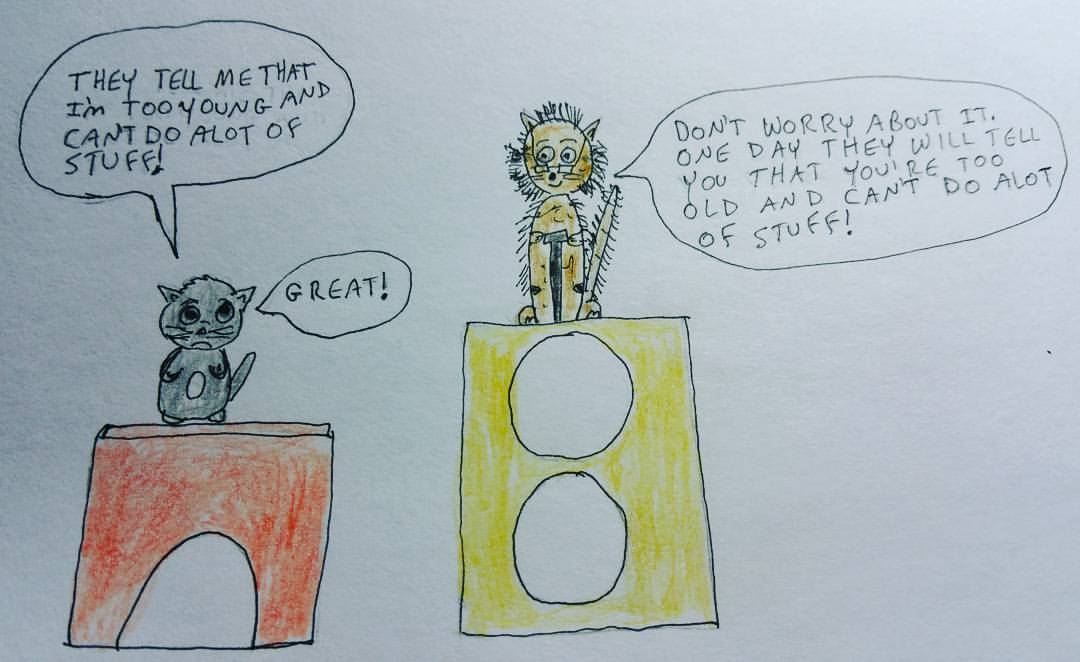In this hand-drawn cartoon image, set against a predominantly white but dark-hued background, we see two main characters: a gray cat and an older creature, possibly another cat, with sparse, wild hair. The gray cat, positioned on the left side and sitting atop a reddish structure that could resemble a tunnel or stand, expresses frustration with a speech bubble that reads, "They tell me that I'm too young and can't do a lot of stuff." To the right, higher up on a yellow rectangle with two white circles, stands the older, yellowish creature with a smirk on its face. This figure reassures the young cat by saying, "Don't worry about it. One day they will tell you that you're too old and can't do a lot of stuff." The young cat, now frowning, responds with a simple, disheartened "Great." The colors in the image primarily include shades of black, white, gray, orange, and yellow, and the overall style suggests a whimsical, yet insightful, artwork that might have been drawn by a child or young adult.